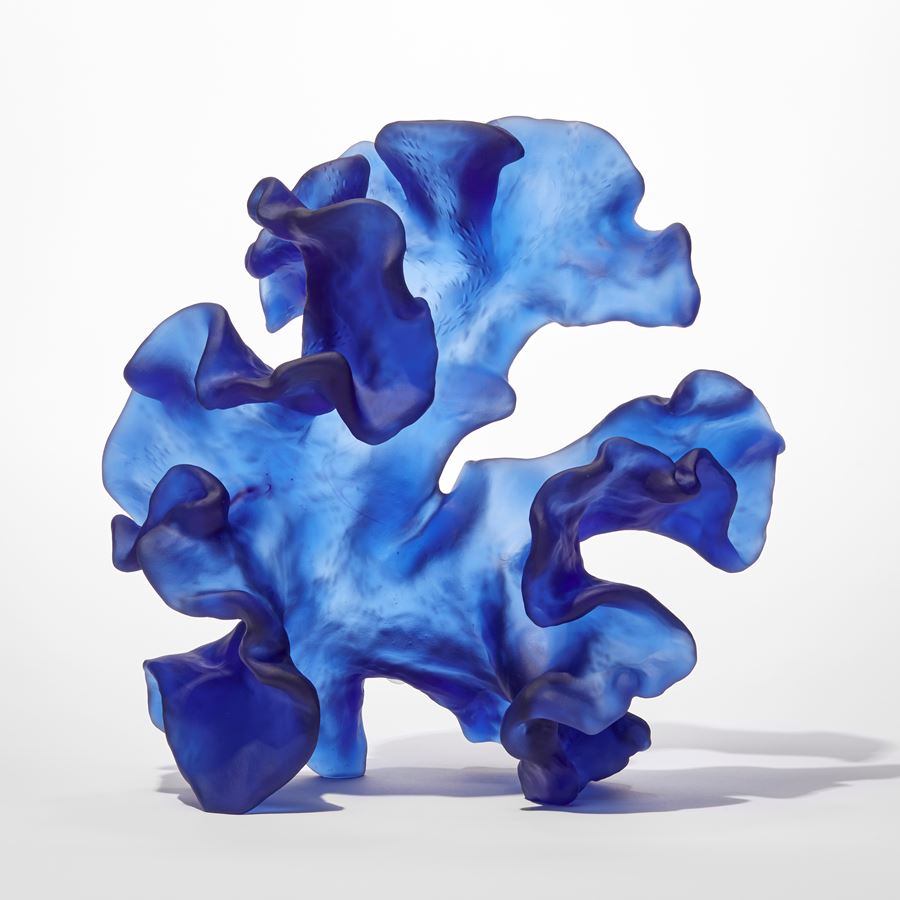The image depicts a semi-transparent, abstract blue glass sculpture that evokes the appearance of a rumpled piece of fabric or a flower petal. The rectangular object, slightly shorter on the top and bottom sides compared to the left and right, appears to float in an empty white void due to a solid white background and surface. The lighting from the top left corner casts a subtle shadow behind and to the right of the sculpture, reinforcing its delicate, almost weightless presence. The glass material combines light and dark blue hues, with intricate curves and lines that give it an organic, fluid form, further enhancing its ethereal, almost otherworldly aesthetic.